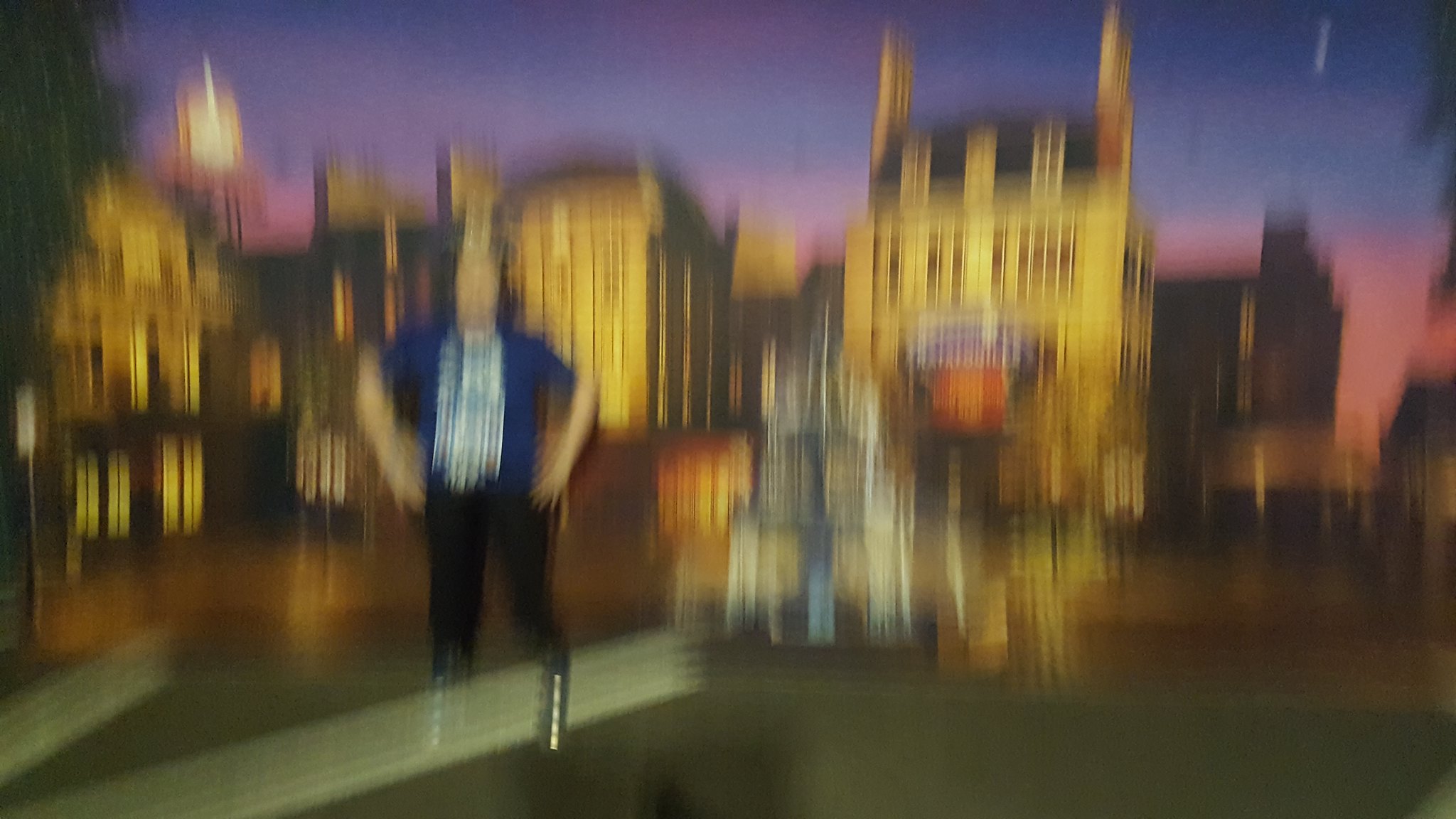The photograph appears to be a highly blurred image of a person standing on a stage, possibly for a theater production or comedy show. The individual, likely a man, is wearing black pants, shiny black boots, and a blue shirt with a blue vest over a white undershirt. They have long black or dark brown hair and are posing with their hands on their hips, arms spread out. The stage has a dark gray floor with white spotlighting that casts shadows over their legs. The backdrop features an image of a cityscape at night, which looks like an older European city with illuminated buildings that have yellow tones, towers, and dormers. The skyline transitions from a blue to pink hue, indicating a late sunset. Trees can be seen off to the left side of the backdrop, adding to the scenic setting.